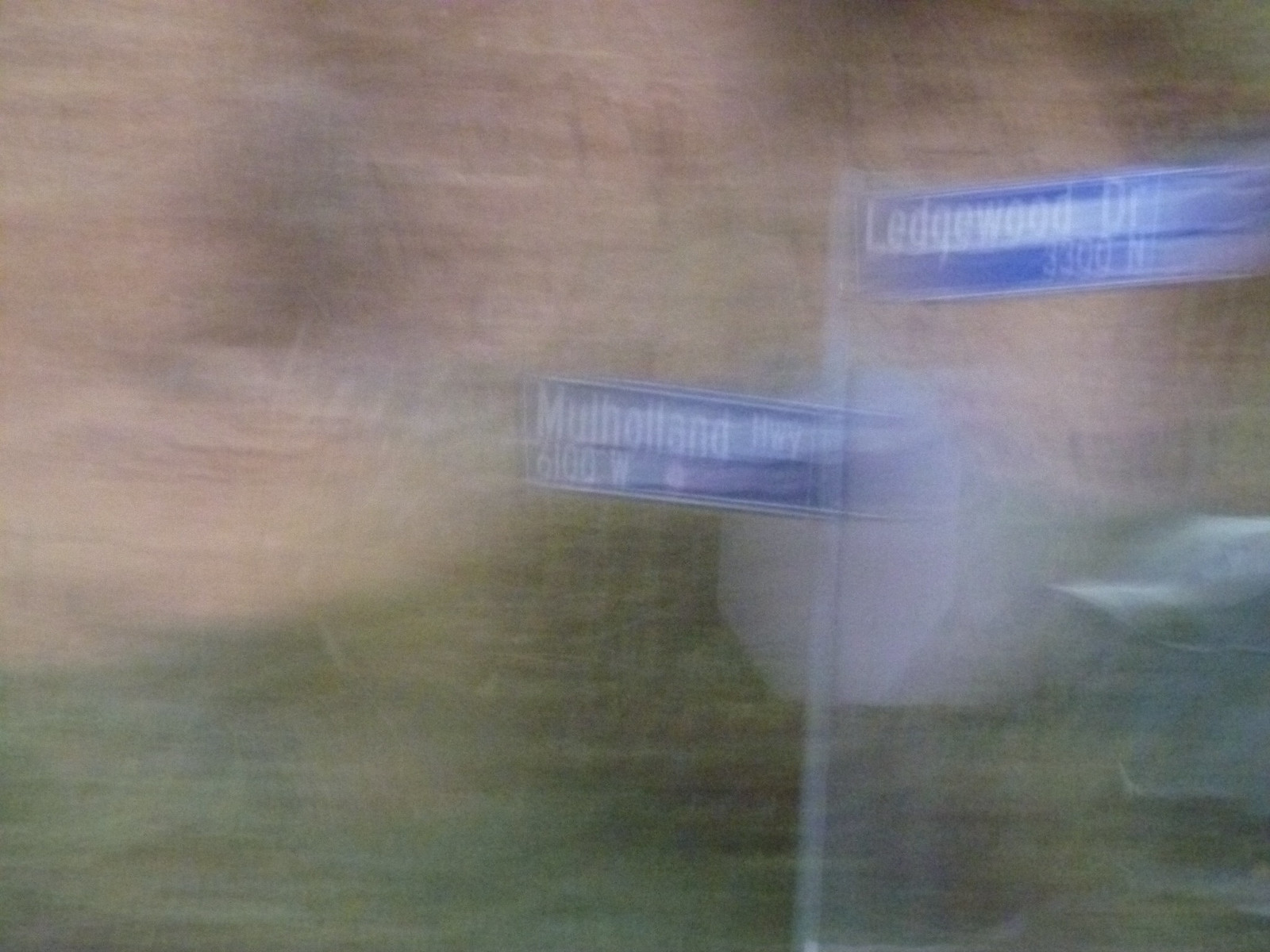This photograph, likely taken from within a car through a foggy window, is not very clear and appears hazy. The image captures a street sign pole and a stop sign. The top street sign, in blue, points to the right and reads "Ledgewood Drive 3300 North." Below it, another sign points to the left and indicates "Mulholland Highway 6100 West." The back of a stop sign is also visible, angled slightly away. The upper section of the photo has a flesh-colored hue, transitioning to green below, suggestive of a reflection, possibly of the photographer's skin, on the car window.